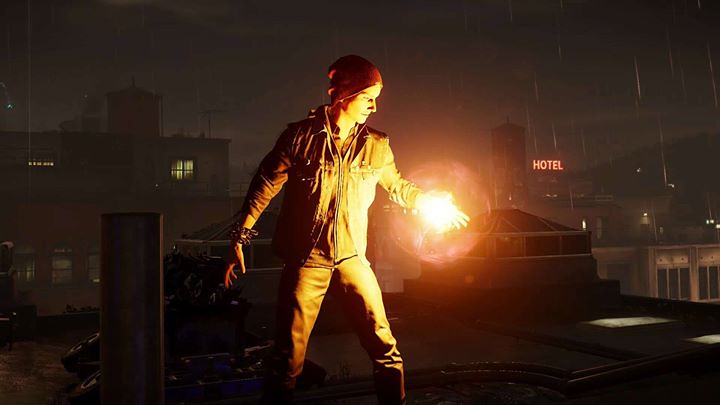A horizontal image captured from a computer screen depicts a figure standing in an urban nightscape. The figure, clad in a long-sleeved denim jacket and collared shirt, pairs the outfit with leather pants. Bathed in a reddish-yellow hue attributed to the nighttime setting, the figure holds a bright white light in their open left palm. This light, encircled by a glowing halo, illuminates the figure in warm tones. The cityscape in the background features a variety of buildings, with some windows lit up. To the right center, a neon red "HOTEL" sign stands out against the otherwise dark, black sky. The figure, wearing a red stocking cap, is positioned centrally in the image, captured from mid-calf upwards to just above the head.